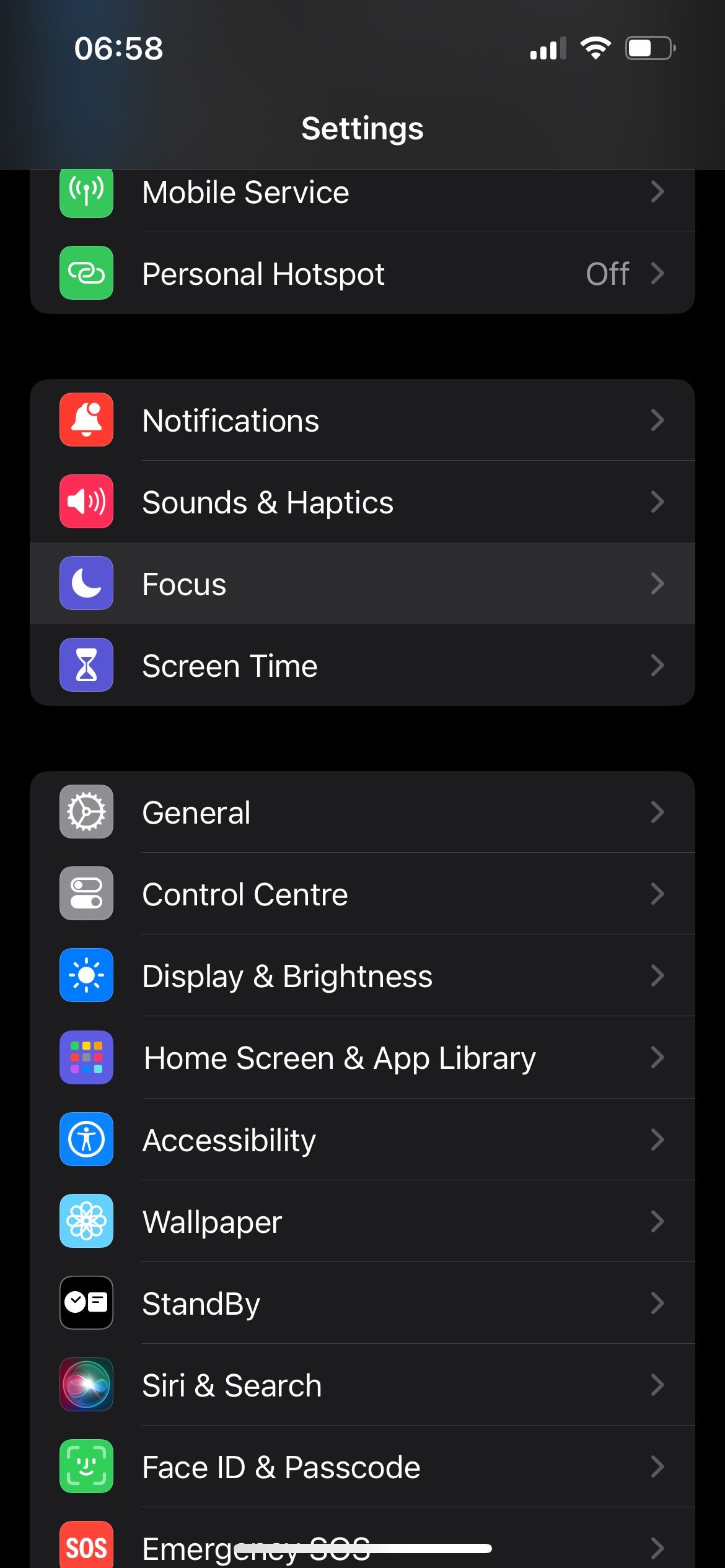The image depicts a mobile phone's settings screen with a black background and white text. A thin white bar extends about one-third across the bottom portion of the screen, partially obscuring the "Emergency SOS" option, which features a red square icon with "SOS" in white text. Each settings option is accompanied by a small right-facing arrow. 

At the top center of the screen is the word "Settings." Listed options include:
1. **Mobile Service** - Identified by a green icon.
2. **Personal Hotspot** - Displayed with a green icon and noted as turned off.
3. **Notifications** - Marked with a red icon.
4. **Sounds & Haptics** - Represented by a red icon.
5. **Focus** - Indicated by a blue icon featuring a white moon.
6. **Screen Time** - Depicted with a blue icon showing an egg timer.
7. **General** - Signified by a grey icon.
8. **Control Center** - Shown with a grey icon containing bar elements.
9. **Display & Brightness** - Labeled with a blue icon featuring a sun in white.
10. **Home Screen & App Library** - Noted by a blue icon with multicolored dots.
11. **Accessibility** - Illustrated with a blue icon including a white circle.
12. **Wallpaper** - Represented by a light blue icon with a white petal design.
13. **Standby** - Featured with a black and white icon.
14. **Siri & Search** - Denoted by a blurred multicolored circle icon.
15. **Face ID & Passcode** - Highlighted with a green icon.
16. **Emergency SOS** - As previously mentioned, it stands out with an SOS label in white on a red icon.